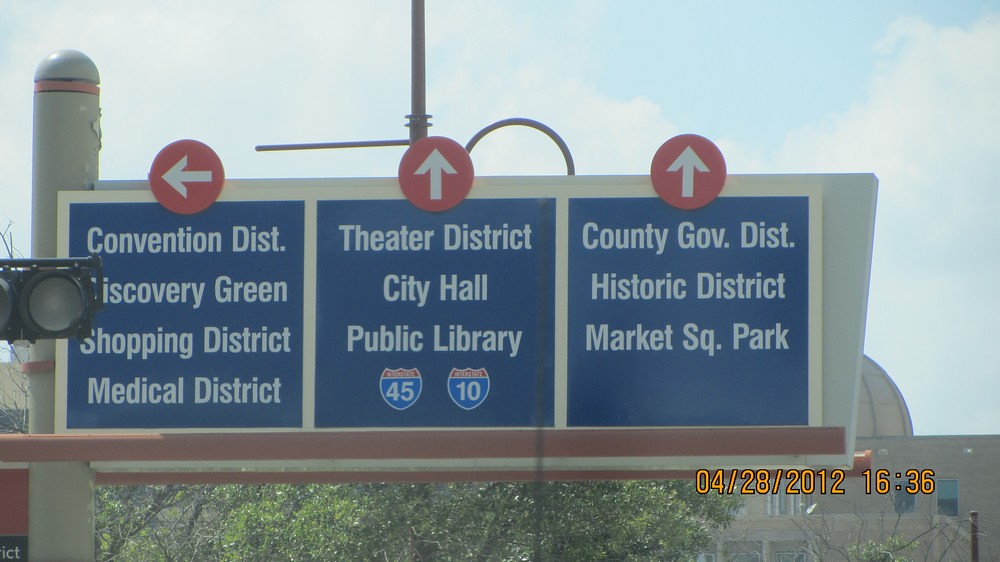The image captures a directional street sign in a city, divided into three sections framed in white with a blue background. Each section features distinct white text and red arrows indicating different directions. The left section, with an arrow pointing left, directs to the Convention District, Discovery Green, Shopping District, and Medical District. The middle section, with an upward-pointing arrow, guides to the Theater District, City Hall, Public Library, and highways 45 and 10. The right section, also with an upward-pointing arrow, leads to the County Government District, Historic District, and Market Square Park. A timestamp reading "04-28-2012 16:36" is visible in the lower right-hand corner of the image, partially concealing a building in the background. Trees and a traffic light are also present, and the sign is mounted on a post against a backdrop of blue sky and white clouds.